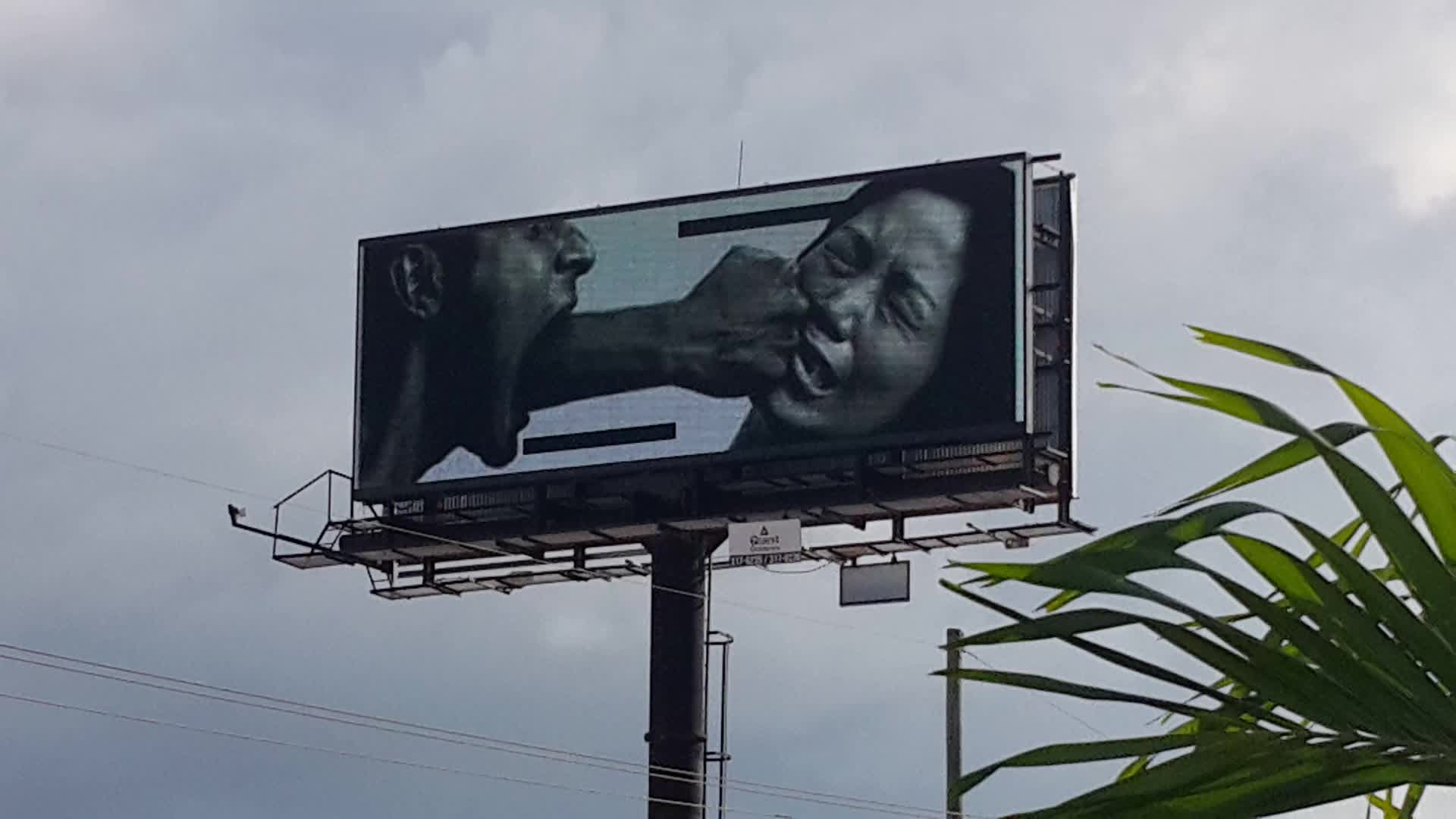In the photograph, a billboard stands tall against a cloud-covered gray sky. Positioned in the lower right corner of the frame, a green leafy plant that resembles a palm frond adds a touch of color to the otherwise monochromatic scene. The rectangular billboard itself is rendered entirely in black and white. On the left side of the billboard, a man's face is depicted with his mouth wide open in a scream. An arm extends from his mouth, ending in a clenched fist that is striking a woman on the right-hand side of the billboard. The woman's face contorts in pain, her eyes tightly shut and her head snapping back from the force of the punch. Her mouth is partially open, showing the intense discomfort she experiences. The stark image is devoid of any text, with two black bars suggesting where words might have been.